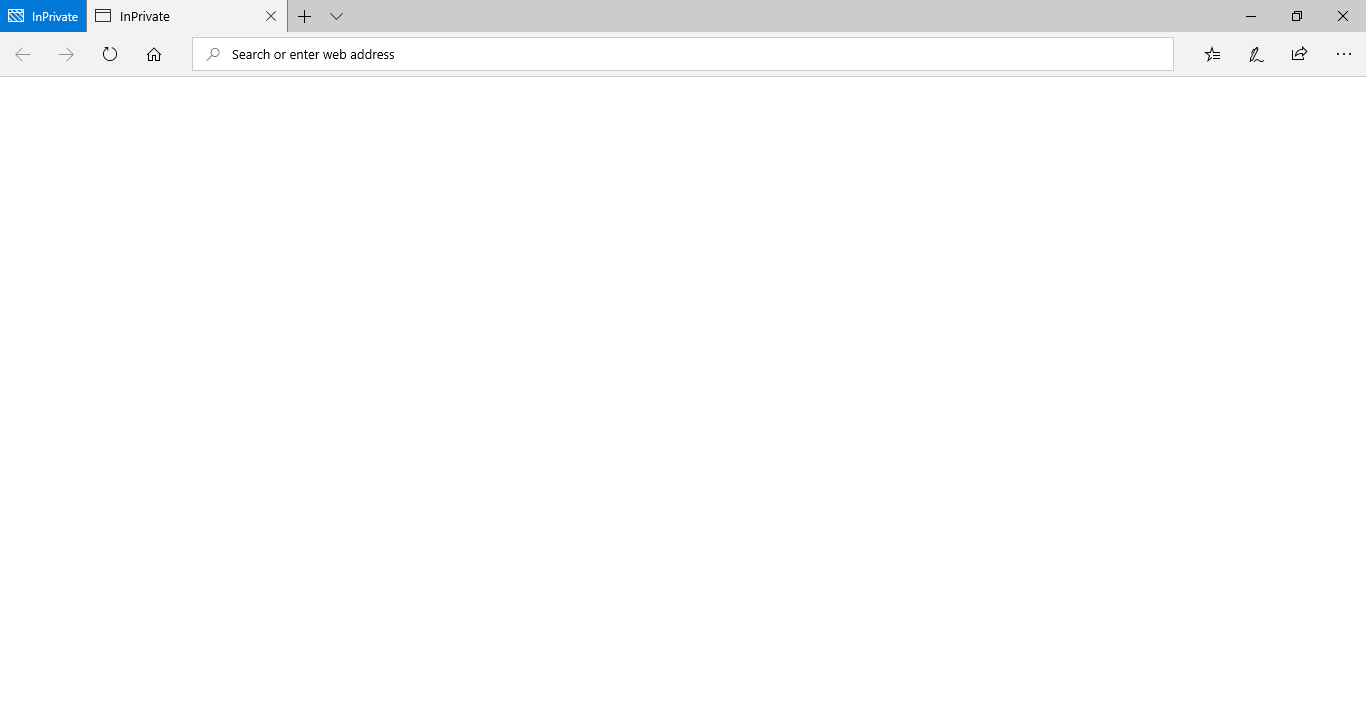The image depicts a completely blank web browser window. At the very top of the browser, there are the usual window control icons – a minimize button, a maximize/restore button (represented by two overlapping squares), and a close button (represented by an "X"). Below that, the browser has a tab bar with an active tab that appears blue, indicating it is in private browsing mode.

Directly underneath the tab bar is the navigation bar. On the far left, there is a home icon followed by a reload button (depicted as a circular arrow). Next to these, there are left and right arrows for navigating backward and forward through web pages. In the center of the navigation bar, there's a search bar that contains a magnifying glass icon and the placeholder text, "Search or enter web address." To the right of the search bar, icons for bookmarks (a star), a pin, an arrow pointing to the right (possibly for sharing), and a menu represented by three vertical dots are visible.

The rest of the webpage is completely blank, indicating no content has been loaded or displayed. The simplicity of the page suggests it might be a new tab page awaiting user input.